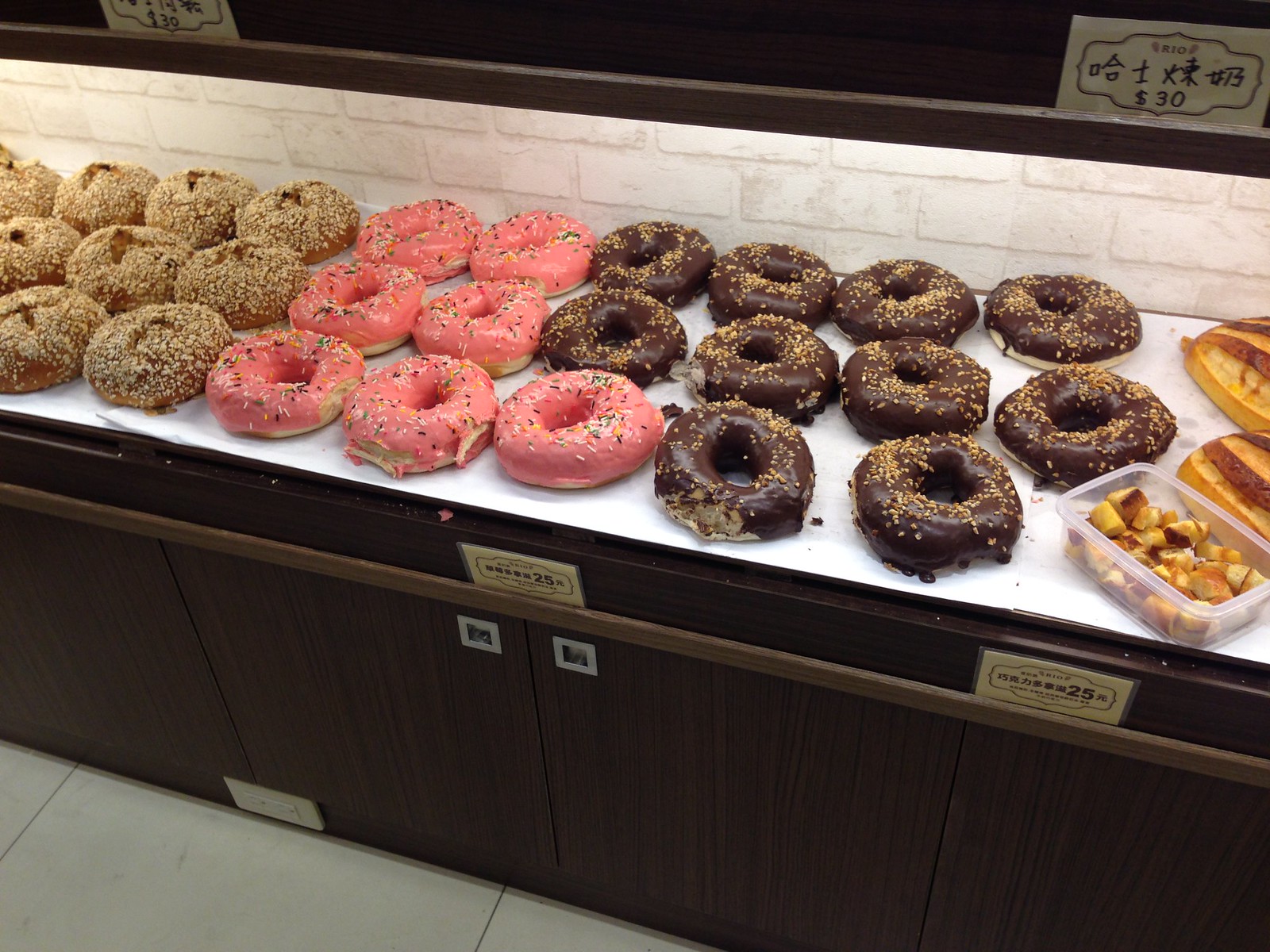This photograph depicts a display at a bakery, most likely a donut shop, showcasing a variety of baked goods arranged on a light, off-white tiled table covered with a white piece of parchment paper. Starting from the left, there's a selection of large, round pastries coated in crushed peanuts or nuts, which appear brown in color. Next to these are donuts with a pink glaze, reminiscent of ones popularized by the character Homer Simpson, complete with colorful sprinkles on top. Following this are chocolate-glazed donuts adorned with gold-colored sprinkles or seeds. In the upper right-hand corner of the image, there's a small white sign featuring foreign characters, which could be Korean, and a dollar sign indicating '30'. On the far right, the display includes additional items such as cut-up bread in a plastic bin and some larger bread loaves, rounding out the assortment of delicious treats.